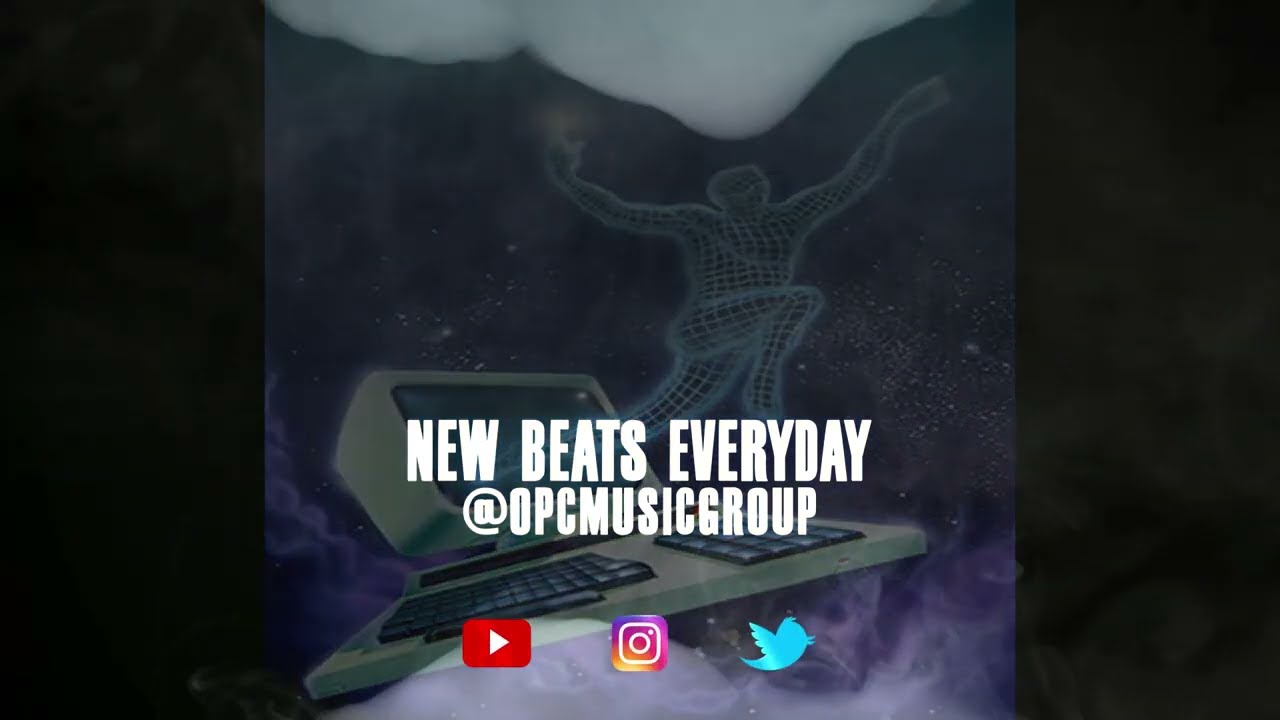The image features a dynamic advertisement for OPC Music Group with the bold, block lettering "New Beats Every Day at OPC Music Group" prominently displayed in the center. Below this text, there are three social media icons: a red square with a white play button symbolizing YouTube on the left, the Instagram logo in the middle, and the Twitter logo on the right. The background is predominantly black, accented with wispy smoke floating up from the bottom. It also incorporates an intriguing visual of a figure composed of white grid lines against a black backdrop, appearing to leap or run with arms outstretched and one leg up. This figure seems to be emerging from an old-fashioned computer with a white keyboard and a small screen, which is positioned amidst a cloud-like formation at the top. The sides of the image are framed by bold, black borders, emphasizing the central content.